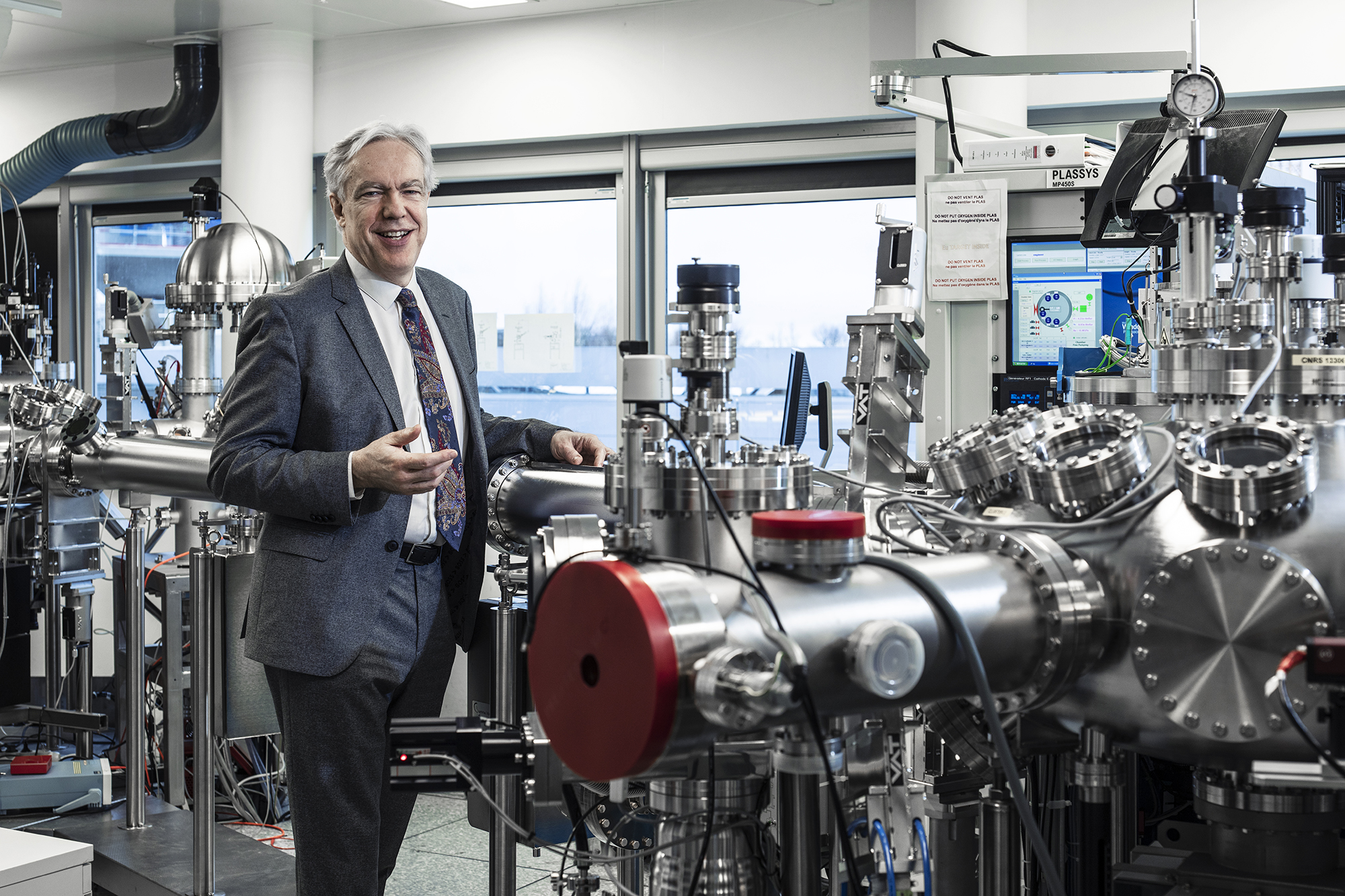The image depicts a man in his sixties with gray hair standing inside what appears to be a laboratory or factory filled with sophisticated machinery. He wears a dark gray suit with matching pants, a white button-up shirt, and a dark purple-black tie adorned with small floral patterns. He is slightly off-center to the left, smiling warmly at the camera. His right hand rests on a part of the silver machinery, which features cylindrical shapes, bolted sections, and circular domes with red caps. His left hand is raised in a friendly greeting gesture. The background reveals various digital screens displaying diagrams, a couple of papers pinned to the wall, and a window with a view to the outdoors. Additional silver tubes, cylinders, and fittings are visible on both sides of the image, emphasizing the industrial and scientific environment.